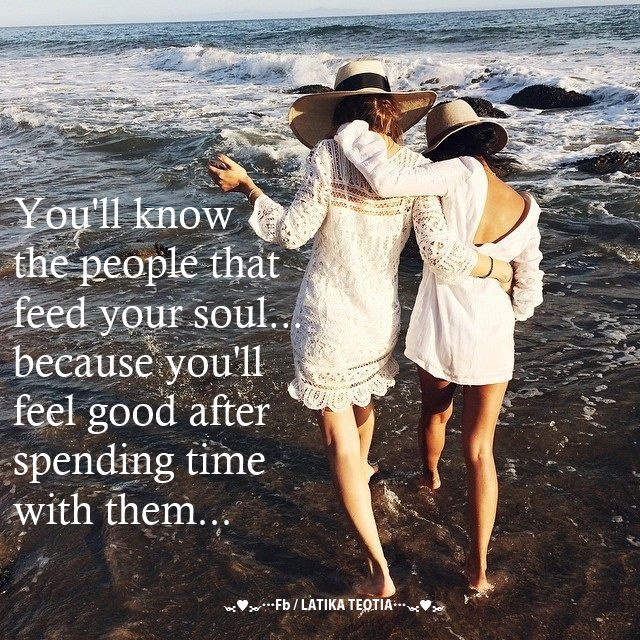The image depicts two women walking hand-in-hand along the shoreline, where the gentle ocean waves lap at their feet. Both women are dressed in knee-length, flowing white beach gowns and don wide-brimmed straw hats that shield their peach-toned faces from the mid-afternoon sun, which appears to be setting in the horizon, casting a warm glow. The woman on the left is slightly taller and has her right arm wrapped around the waist of the woman on the right, who has her left arm draped over her companion's shoulder. They walk on flat rocks partially submerged in the shallow water, with waves breaking against higher rocks in the background. The scene is serene, with calmer waters beyond the crashing waves. On the left side of the image, a quote in white text reads, "You'll know the people that feed your soul... because you'll feel good after spending time with them," attributed to Facebook user Latika Teotia.